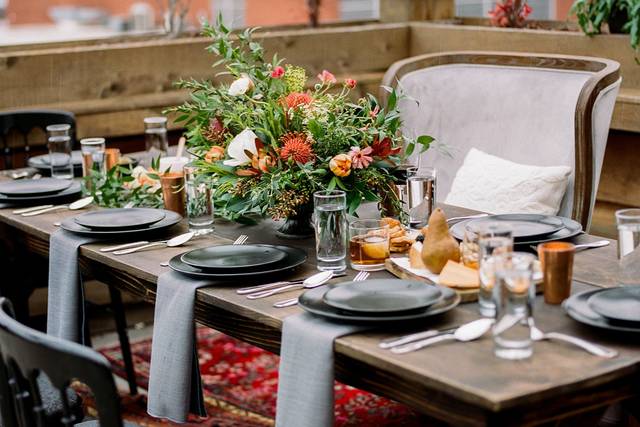This photo captures a meticulously arranged outdoor dining setting with a long rectangular dark wood table set for 10. The arrangement boasts 10 black and shiny plates, each paired with a smaller plate on top, accompanied by gray linen napkins hanging down beneath. Silverware is neatly positioned on either side of the plates, and the table is adorned with tall glasses of water and some alcohol glasses. The detailed centerpiece comprises a bouquet of various flowers in shades of orange, red, and white, contributing to the elegant ambiance. The setting includes an array of chairs, notably a white chair with a cushion on one side and a black chair on the other, along with a chair in the background with a wood exterior and a pillow. A board with pears and cheese adds a touch of rustic charm, while a red carpet underneath the table ties the scene together. The backdrop reveals buildings and plants, confirming the outdoor locale, and the overall appearance is professionally arranged and inviting, with no people in sight.